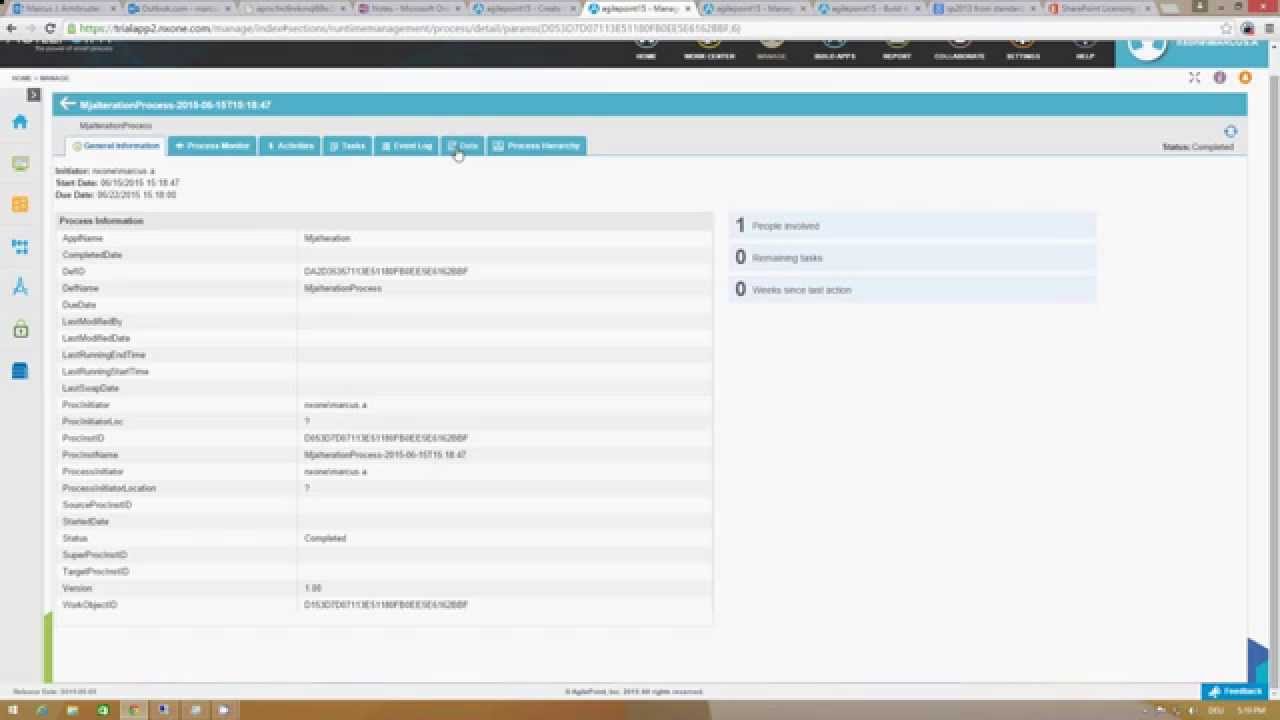The image appears to be a screenshot of a computer screen displaying a web browser with several open tabs displayed along the top bar. Below the tabs, there is an indistinct website currently active, though the text is not legible. Beneath the website header is a prominent blue navigation bar, followed by a series of clickable blue rectangles, one of which is being selected by a white cursor resembling a pointing finger, likely indicating an active button, possibly labeled "Home" or similar. The central portion of the screen shows a structured layout with alternating gray and white lines containing unreadable black text. Along the left side of the page, these gray and white lines continue in a similar pattern, all filled with text. At the very bottom of the screenshot is a brown taskbar featuring various clickable icons, including one reminiscent of the Google Chrome logo.